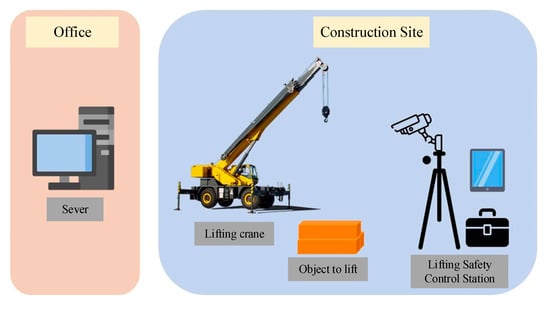The image consists of two distinct sections. On the left, a smaller image features a pink salmon-colored background with the label "office." This section contains a pixelated picture of a computer monitor and tower, captioned "server." To the right, a larger image with a pale blue background is labeled "construction site." At the top, it showcases a yellow crane with the tag "lifting crane." In the bottom center, there's a stack of three orange items labeled "object to lift," indicating these are the items the crane is meant to lift. Further right, a camera on a tripod, a tablet-like screen, and a black handled case are collectively labeled "lifting safety control station." The detailed juxtaposition of these elements highlights the contrast between an office environment and a construction site, focusing on equipment and safety mechanisms.